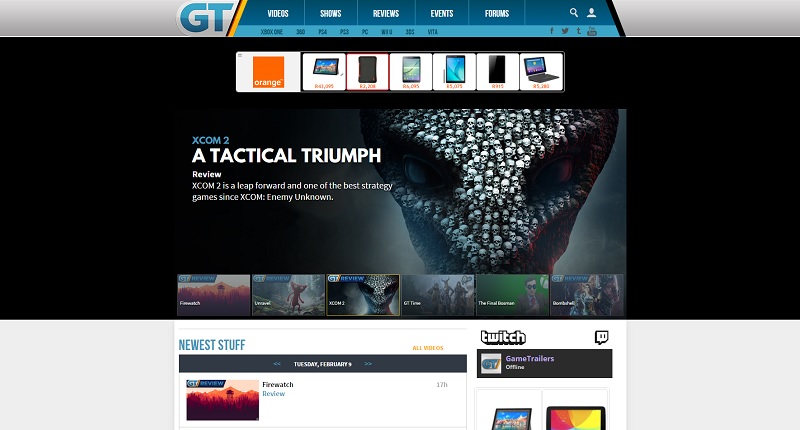This is a cropped screenshot of a website known as GT. The header is light gray, with an angled yellow bar positioned slightly to the left. To the right of the yellow bar are five categories: Videos, Shows, Reviews, Events, and Forums. Below the header, there is a lighter blue line that features another set of five categories extending across the screen. 

Directly beneath this line, an advertisement with a prominent 'X' in the top left corner displays thumbnails showcasing various electronics. Following the advertisement, there is a striking large image that depicts an alien head covered in crystals or potentially composed of multiple smaller alien heads. To the left of this intriguing image, 'XCOM 2' is written in small blue letters, with the caption 'A Tactical Triumph' in large white letters below it. Further down, 'A Review' is indicated in smaller white lettering.

At the base of the image, six thumbnails are visible, with the third thumbnail being selected, indicating its display on the background. The bottom left corner of the screen prominently features the text 'NEWEST STUFF' in bold capital letters. Adjacent to this, 'Twitch' is noted, followed by the account's name on the Twitch platform.